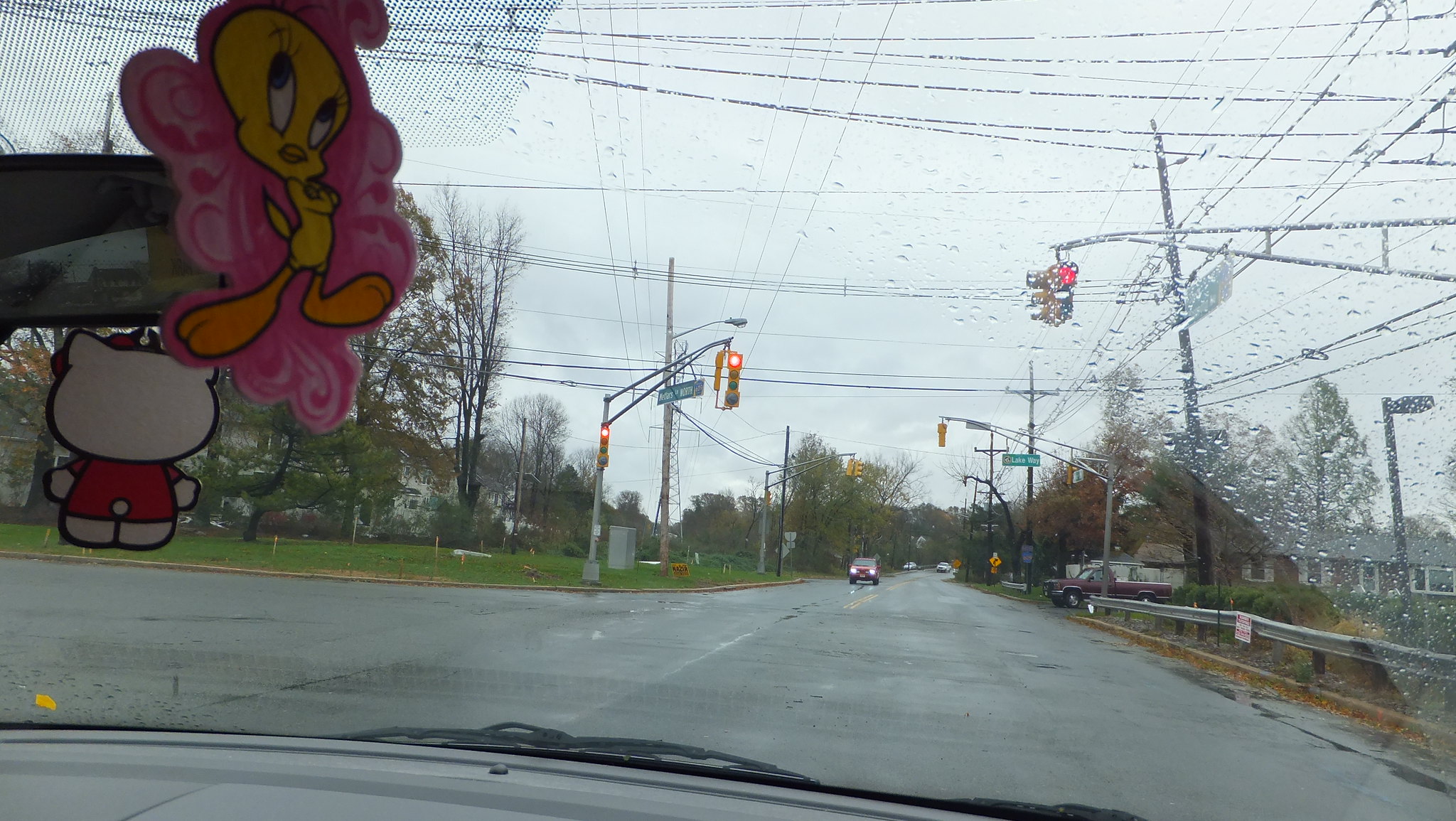Captured from the interior of a car, this street scene photograph artfully combines the dynamic elements of both the inside and outside environments. Raindrops speckle the windshield, creating a naturally occluded view beyond, though a streak of clarity hints that the windshield wipers have just swept through. Through the windshield, a four-lane street stretches forward, with only a couple of cars faintly visible in the distance. A stoplight hangs prominently, signaling to the driver, and directional signage indicates the street names.

On the right side of the street, a curb and a protective metal barrier highlight the attention to road safety. Far in the distance, homes and a truck are discernible within the flat landscape, adorned with bare trees and patches of grass on the opposite side of the street.

Inside the car, a few personal touches add a sense of coziness and aroma to the scene. A charming Tweety Bird decoration, surrounded by pink embellishments, dangles invitingly. Another figure, resembling the back of a small bear or cat, also hangs from the rearview mirror, likely serving as a fragrant ornament to enhance the car's interior ambiance. Overall, the image captures a transient moment of everyday life, enriched by the interplay of weather, surroundings, and personal comfort.